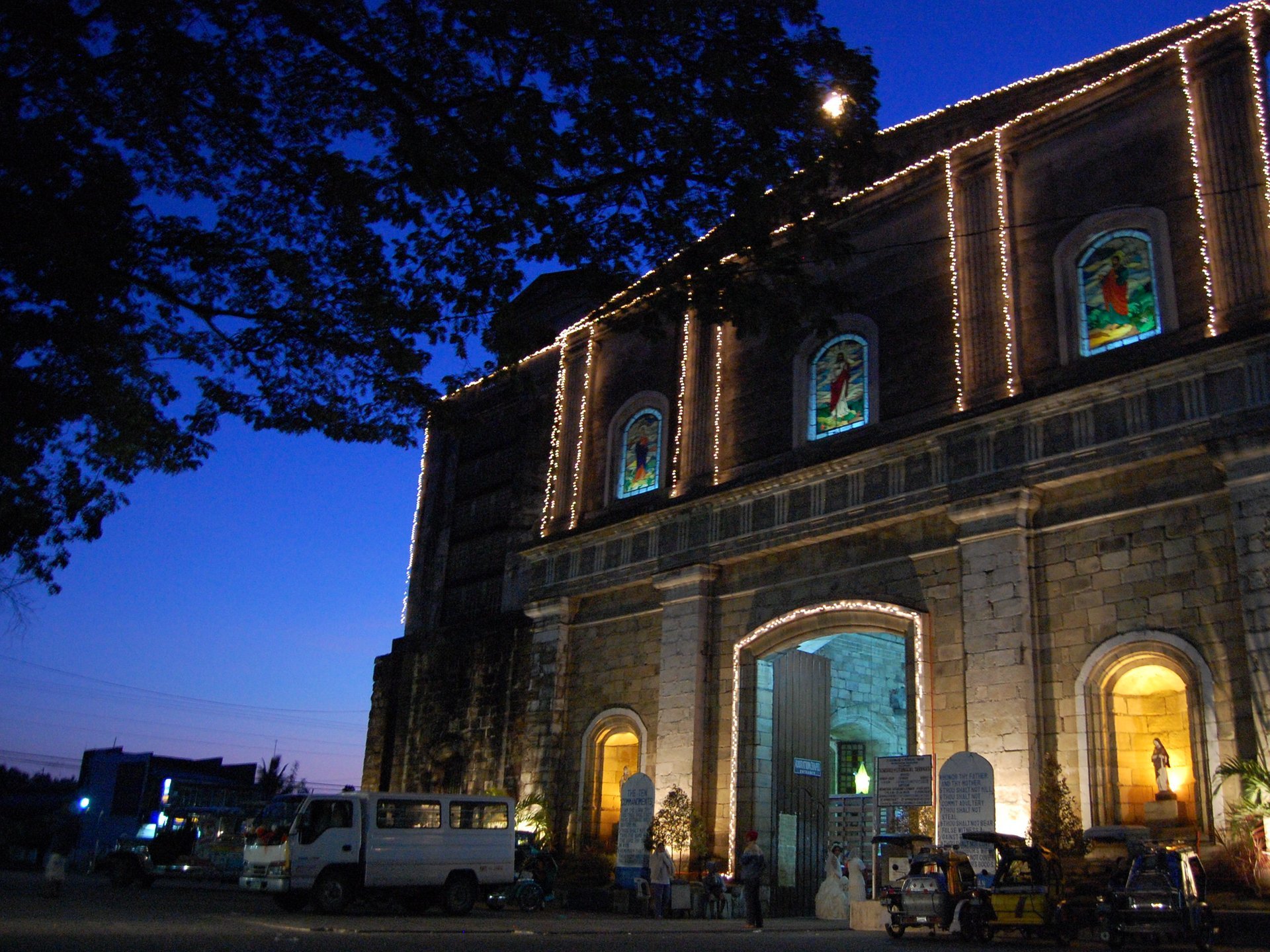The photograph showcases a large, imposing cathedral built from light brown stone, set against a darkening evening sky tinged with hues of deep blue and purple. The cathedral has a grand facade featuring three tall, elaborately detailed stained glass windows on its upper story. The central window depicts Jesus Christ, flanked by windows of Mary on the left and an unknown saint on the right. Illumination from inside casts a soft blue light through the central archway, creating a captivating nighttime scene. Recessed niches on the lower level house statues of the Virgin Mary, glowing with golden yellow light. String lights further embellish the upper part of the building. 

In front of the cathedral, the street is populated with various vehicles, including a large white van on the left and a series of smaller cars to the right, along with a truck further to the left. The cathedral’s towering doors stand wide open, revealing a couple of people near the entrance, one of whom appears to be wearing a wedding dress. A lighted star mounted on a stick and several stone markers or signs add to the scene's details, while a silhouetted tree branch and leaves partially frame the upper left corner.